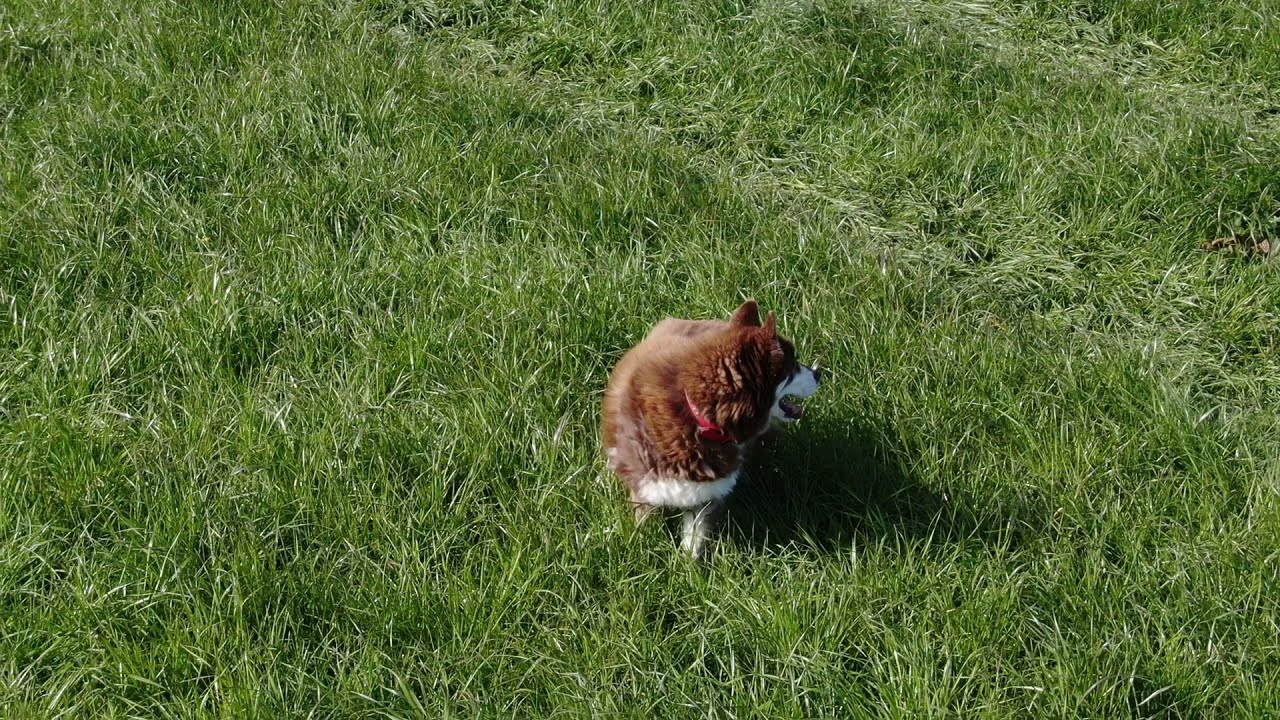This is a daytime photograph featuring a small brown and white dog standing in the middle of a grassy area. The dog's upper body is predominantly brown, while its lower body, snout, belly, and front legs are covered in white fur. It sports a red collar, seemingly with some writing that is not legible in the image. The dog is captured looking to its right, almost behind it, with its shadow falling to the right side on the lush, wavy green grass, which appears slightly unkempt. The grass dominates the image, surrounding the dog entirely, except for a small trampled patch in the top right corner.